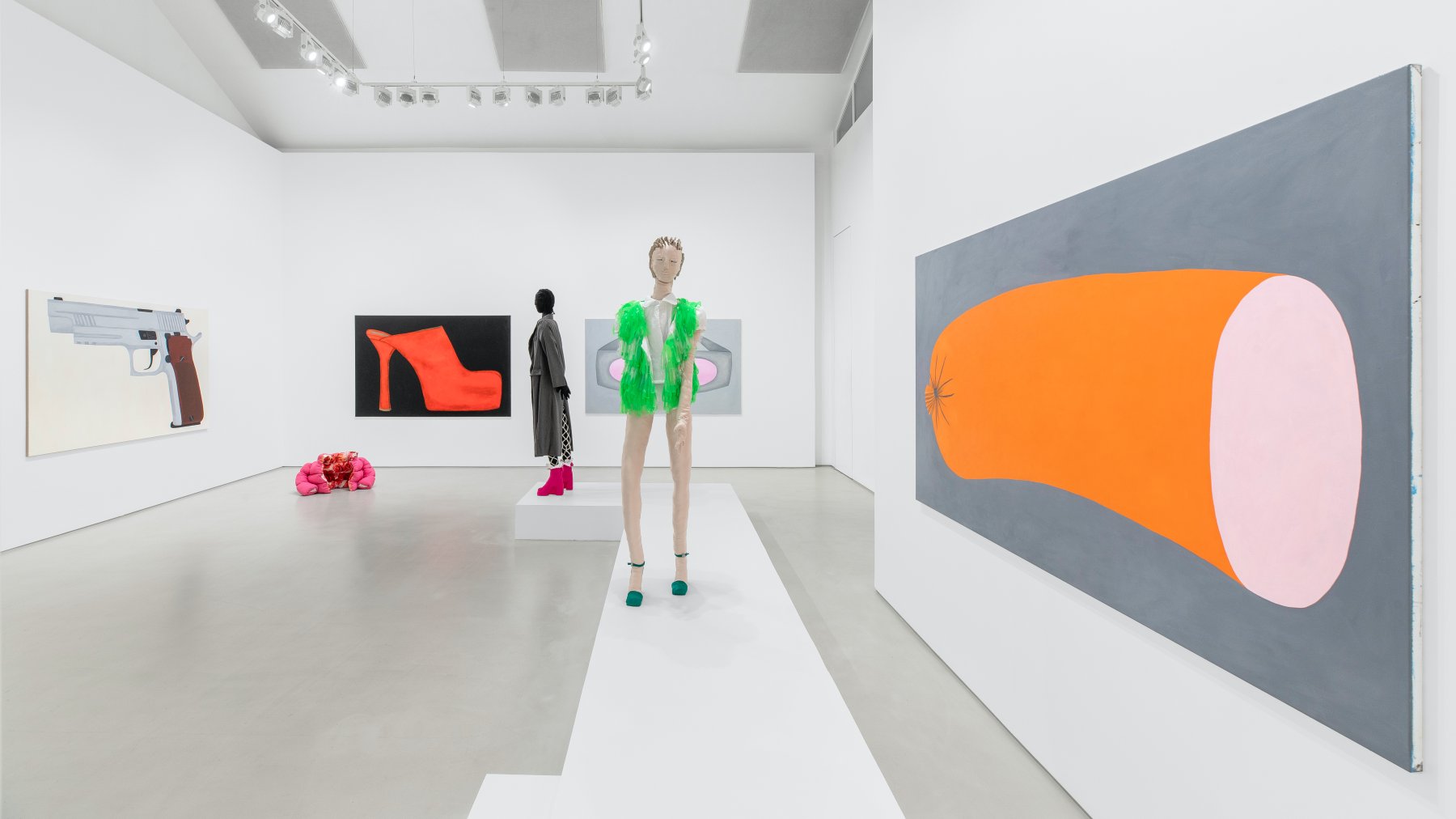This cartoonish model type rendering depicts the interior of a rectangular art gallery with stark white walls and pale grey concrete flooring. Dominating the foreground is a striking mannequin-like figure with elongated legs, dressed in green strappy high heels and a light green short dress over a white shirt. She strides confidently on a white, rectangular runway. To her left, a massive canvas with a greyish-blue background showcases an elongated golden horn figure. In the background, another mannequin stands on the runway, wearing pink boots, a long black trench coat, and a black hood. She gazes at an impressive canvas featuring a pistol with a brown handle.

The gallery contains several other noteworthy pieces. On the right side of the room, a canvas illustrates an orange sausage casing with a pink circle marking the meat portion, set against a grey backdrop. The back wall displays a painting of a red shoe. Near the first mannequin, a somewhat obscured canvas possibly depicts 3D or x-ray glasses. In the left rear corner, a pink chunky sculpture rests on the floor, adding a three-dimensional element to the space. Track lighting from above casts a soft glow over the scene, emphasizing the gallery's meticulous arrangement and the unique artistic creations within it.